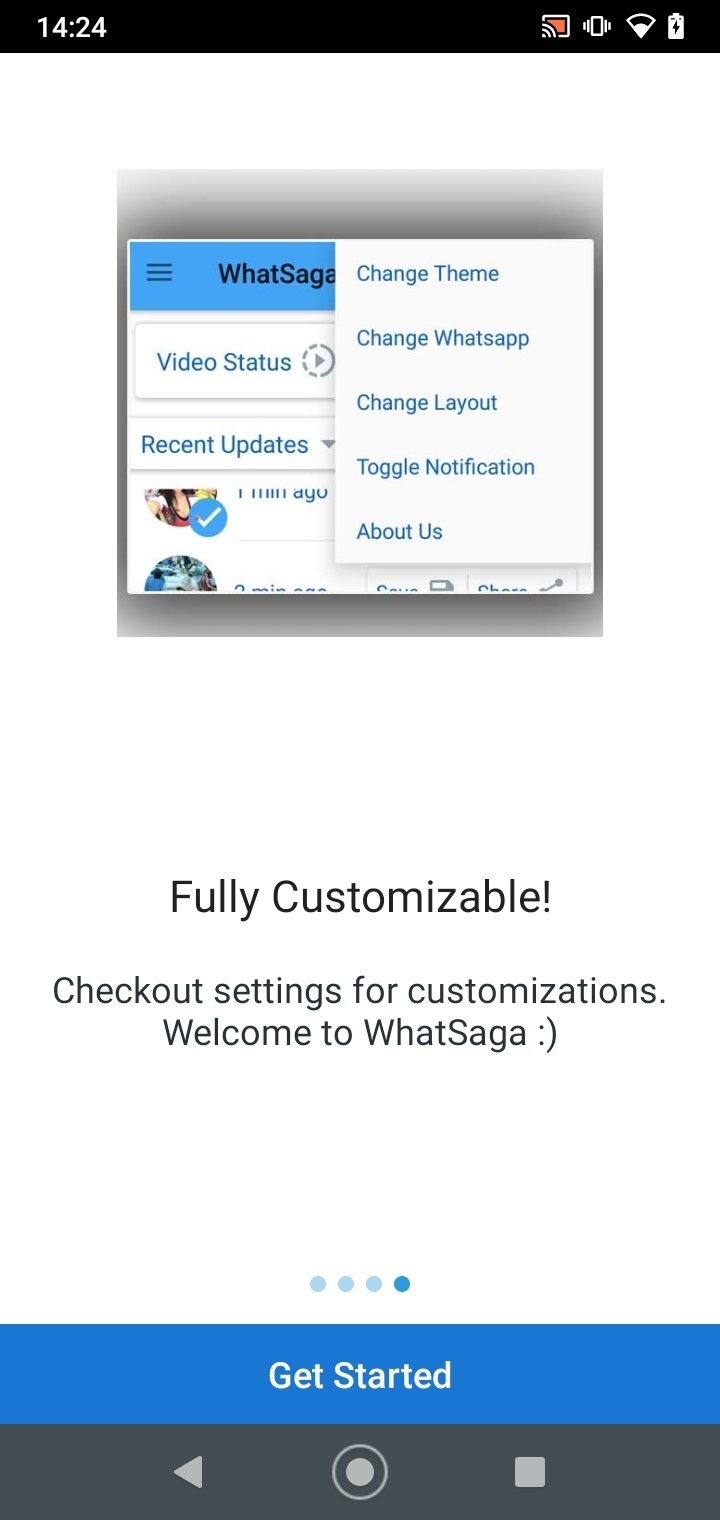The image depicts a screenshot taken on a smartphone. At the top of the image is a black status bar displaying the time as 14:24 in white text. Alongside the time, there are several icons in white: a battery icon indicating it is charging, a WiFi icon, and a sound icon.

Below this status bar is a white background featuring a prominent blue and white pop-up screen. The pop-up contains blue text with various options: "Change Theme," "Change What's Up," "Change Layout," and "Toggle Notification." 

Further down, there is a message in black text stating: "Fully customizable. Check out settings for customization. Welcome to What Saga." Just below this message, there are four light blue dots; the first three are light blue while the last dot is a darker shade of blue, indicating a current selection or active step.

Below these dots is a blue band with the text "Get Started" in white letters. Finally, at the bottom of the image is a black band containing a series of control icons: a play button, record button, and pause button.